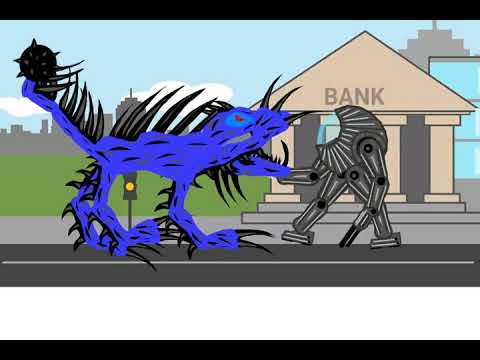The image is a detailed, computer-generated illustration set in a city street marked by a prominent building on the right-hand side labeled "BANK" in gray letters. The bank, characterized by its four beige columns and triangular roof, is situated against a backdrop of a cityscape with shadowed buildings, a blue sky, and white clouds. In the foreground, two animated characters are engaged in a confrontation on the gray road, which features a white center line. On the left stands a blue, dragon-like creature adorned with black and gray spikes along its back, legs, and tail, which ends in a spiked sphere. The creature also has black teeth, a red eye encircled with light blue, and additional spikes near its face and arms. Facing this dragon is a robotic figure described as gray and white with a large, round body, mechanical arms and legs, and a bite-like feature on its head. The street scene is flanked by green grass and a gray sidewalk, with a yellow traffic light visible below the dragon-like creature. The overall illustration merges elements of fantasy and urban environments.